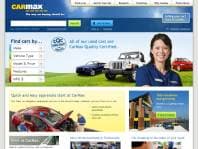The image depicts the homepage of the CarMax website from a distant vantage point. The top banner of the page is a bright blue with the CarMax logo situated on the upper left. The "Car" part of the logo is rendered in yellow uppercase letters, while the "Max" part is in white uppercase letters, both set against a blue background resembling a sky with clouds. 

To the upper right, extending towards the middle, there is a gray-colored menu bar. Below the banner, a dark blue bar features a search bar on the left, with a prominent green button for initiating the search to its right. This bar frames the sky and cloud imagery above it.

Further down, the webpage includes a section that is somewhat difficult to decipher due to its small size. It houses a vertical menu on the left side with five buttons stacked one atop the other. The main visual element of this section shows three cars parked on a grassy hill with a backdrop of sky and clouds. Additionally, a person stands facing the camera in this scene.